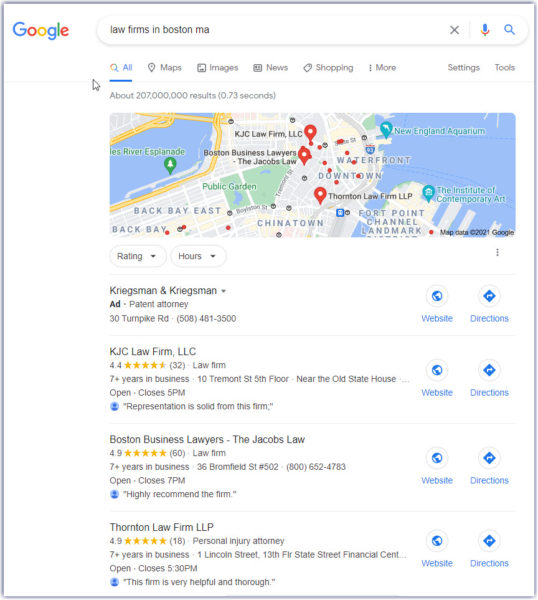Google search result for law firms in Boston, Massachusetts displayed several options, including KJC Law Firm, LLC, which has been in business for over 7 years and holds a 4.4-star rating. The firm is located on the 5th floor near the Old State House and handles business law, patent journeys, and various legal services. Their office at Turnpike Road can be reached at 505-481-2400. Another highlighted option was Zakiya Kosala, a Boston business lawyer with a 4.9-star rating based on 800 votes, located at 36 Palmfield Street. She specializes in business law and her office remains open until 7 pm. Thornton Law Firm, LLP, situated at 1 Lincoln Street in the financial center, also stands out with a 4.9-star rating from 18 reviews. This firm, known for personal injury cases, has over 7 years of experience and closes at 5:30 pm. All these firms display thoroughness and reliability, making them highly recommended within the Boston legal community.